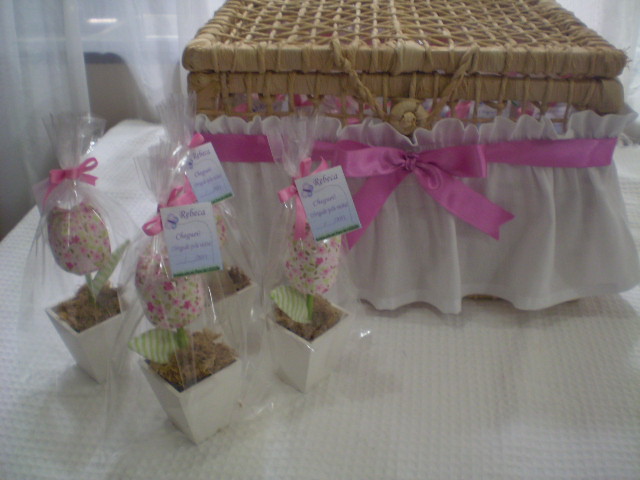This detailed photograph captures a beautifully arranged baby shower gift display featuring a wicker basket adorned with a large pink bow, sitting atop a table draped in a white linen tablecloth. The setting is indoors, framed by delicate white curtains in the background. The basket, covered in a white, delicate skirt-like fabric, sits prominently in the middle of the table. In front of the basket, there are four meticulously crafted edible gifts. Each gift is presented in a small square white pot, filled with brown compost to mimic a plant base. Emerging from each pot are tulip-shaped desserts, artistically speckled with shades of green and pink. These edible tulips are individually wrapped in cellophane and secured with matching pink ribbons, perfectly complementing the pink bow on the basket. Each tulip also features a little card inscribed with the name "Rebecca" in purple writing, though some of the finer details on the cards are slightly blurred. The whole arrangement, with its soft pinks and whites, exudes an air of delicate celebration and thoughtful presentation, highlighting the attention to detail and the festive atmosphere of the occasion.